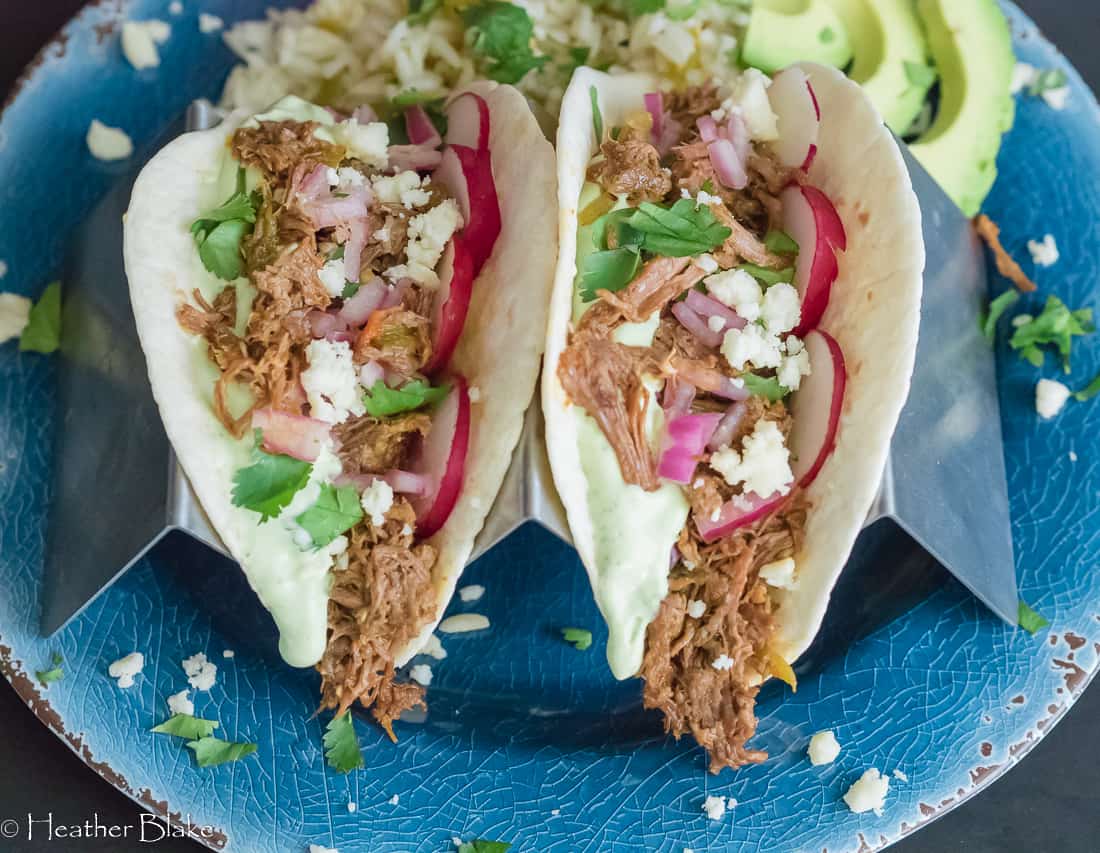This indoor photograph, set in landscape orientation, features a close-up, overhead view of a blue circular china plate holding two tacos. The tacos, nestled in a small metal stand, have flour tortillas filled with shredded pulled pork. Complementing the pork are red onions, sliced radishes, and chopped bell peppers, all topped with crumbles of goat cheese and sprinkles of cilantro. White dots, possibly cheese or corn, scatter across the plate. In the background, slices of avocado and a scoop of white rice with green vegetables, perhaps broccoli, add additional visual interest. The lower left corner bears the text "Heather Blake," marking the photographer's signature. The sides of the plate are partially cut off, revealing a navy-colored background that frames the appetizing scene.